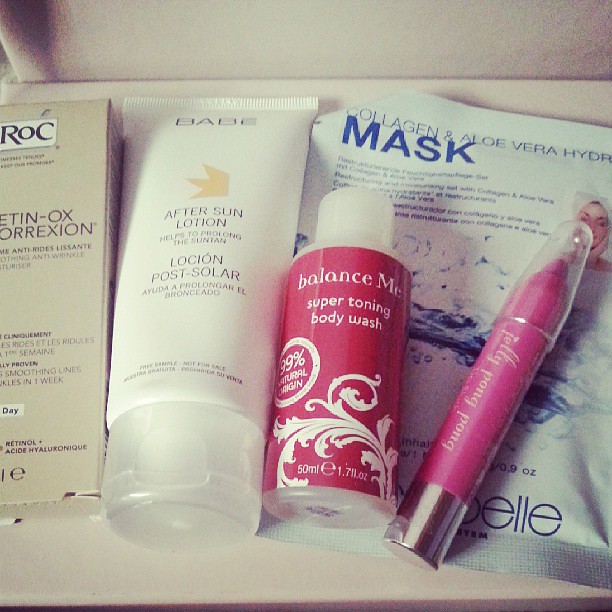The image showcases a collection of beauty and skincare products arranged on a hard, white, flat surface. On the far left, partially cropped out, lies a tan box with black text labeled "ROC" and additional smaller text reading "Retin-Ox Correction," which is difficult to decipher due to size. Next to it is a white tube adorned with blue text that reads "Babe After Sun Lotion," featuring a small yellow flame illustration and promises to help prolong a suntan, with some information also printed in French. Positioned centrally is a small pink bottle labeled "Balance Me Super Toning Body Wash," which claims to be 99% natural origin and contains 50 milliliters. Behind these items, there's a white package displaying blue text for a "Collagen and Aloe Vera Hydra Mask," and an image of a woman wearing the mask. Finally, to the right, there's a pink lipstick pencil or crayon with unreadable text due to the image's slight blur and angle. The entire arrangement appears slightly out of focus, contributing to the difficulty in reading some of the labels.